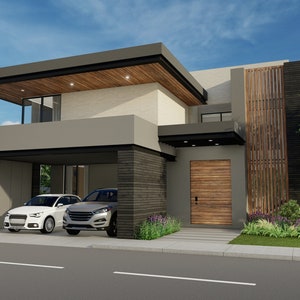The image depicts a modern, computer-generated representation of a house with a distinctly contemporary design. The house features a flat roof with a beige top, a black lining, and a wooden area directly beneath it. The exterior palette combines natural wood tones with gray and white colors, contributing to its sleek and modern aesthetic. 

The structure incorporates a blend of straight edges and clean lines, emphasizing its minimalist appeal. At the left side of the house, there's an open two-car garage housing a white car and a gray truck. The garage lacks a door and seamlessly integrates into the design.

To the right of the garage, there is a prominent wooden front door with a gray frame. Ascending from the door is an arrangement of wooden beams that extend vertically, adding a distinctive element to the facade. Above the entrance, a unique window design includes an overhead wooden section equipped with three lights, enhancing its modern flair.

The top quarter of the image showcases a blue sky with scattered white clouds, creating a pleasant backdrop. Overall, the immaculate detailing of the wooden elements, flat roof, and expansive windows highlights the house's innovative and contemporary style.